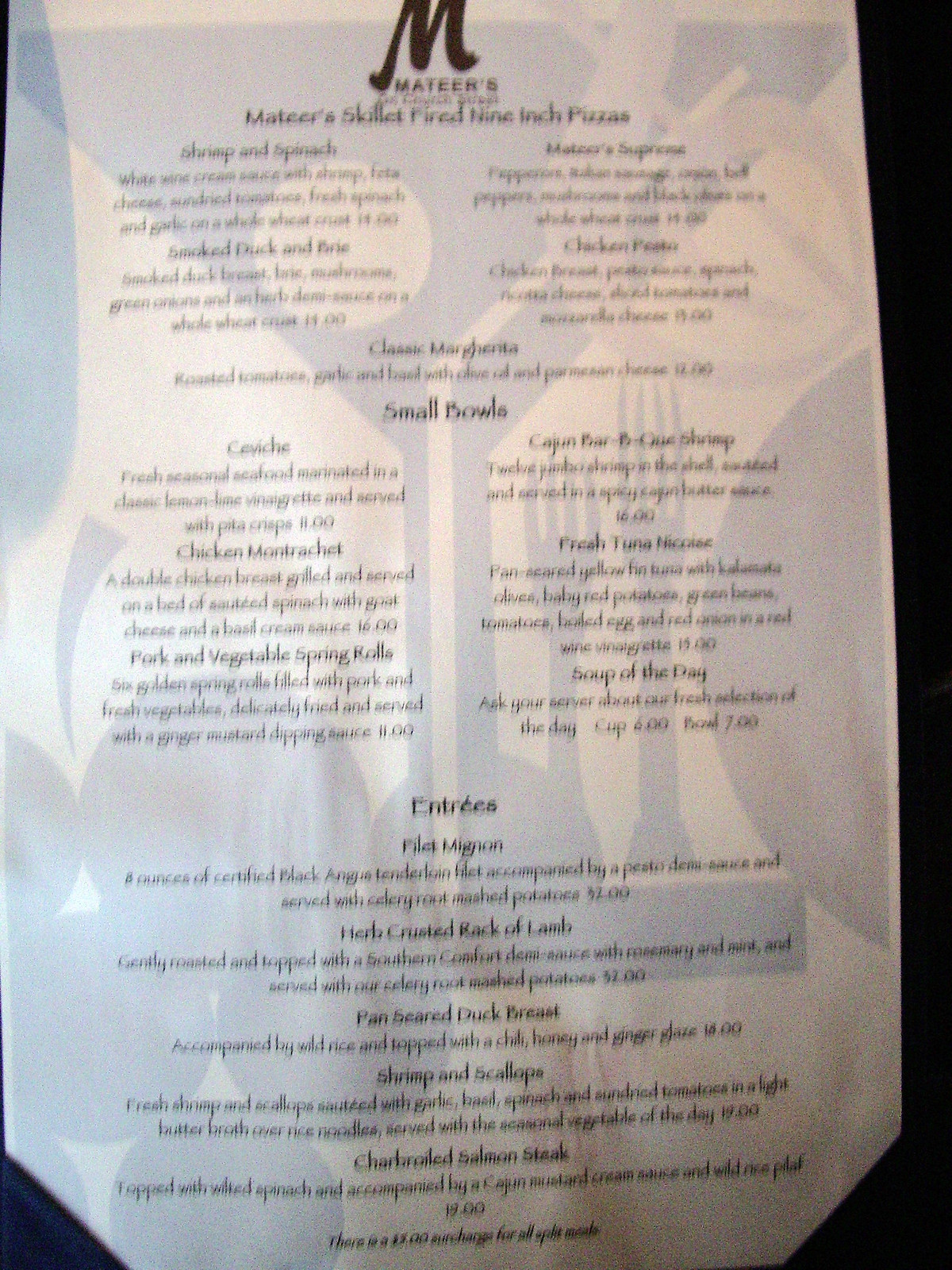Photograph of a restaurant menu with a black background and white paper that features a gray illustration of a wine glass. The menu is artistically designed with various kitchen utensils, including a large fork, a smaller fork, and a partial section of a plate, along with some decorative circles on the left.

At the top, there's a prominent capital letter "M," underneath which "MATEER'S" is written. The menu highlights their skillet-fired nine-inch pizzas with options like Shrimp and Spinach, Smoked Duck and Brie, Chicken Pesto, and a Classic Margherita, each accompanied by detailed descriptions that are unfortunately illegible.

Under the "Small Bowls" section, the first item is unreadable, followed by "Chicken Something" and "Pork and Vegetable Spring Rolls." On the right-hand side, listed items include Cajun Barbecue Shrimp and Fresh Tuna with an unreadable descriptor.

Below this section, the "Entrees" category features Filet Mignon, Herb-Crusted Rack of Lamb, Pan-Seared Duck Breast, Shrimp and Scallops, and Char-Broiled Salmon Steak, each paired with detailed descriptions and prices, most of which are blurred and unreadable.